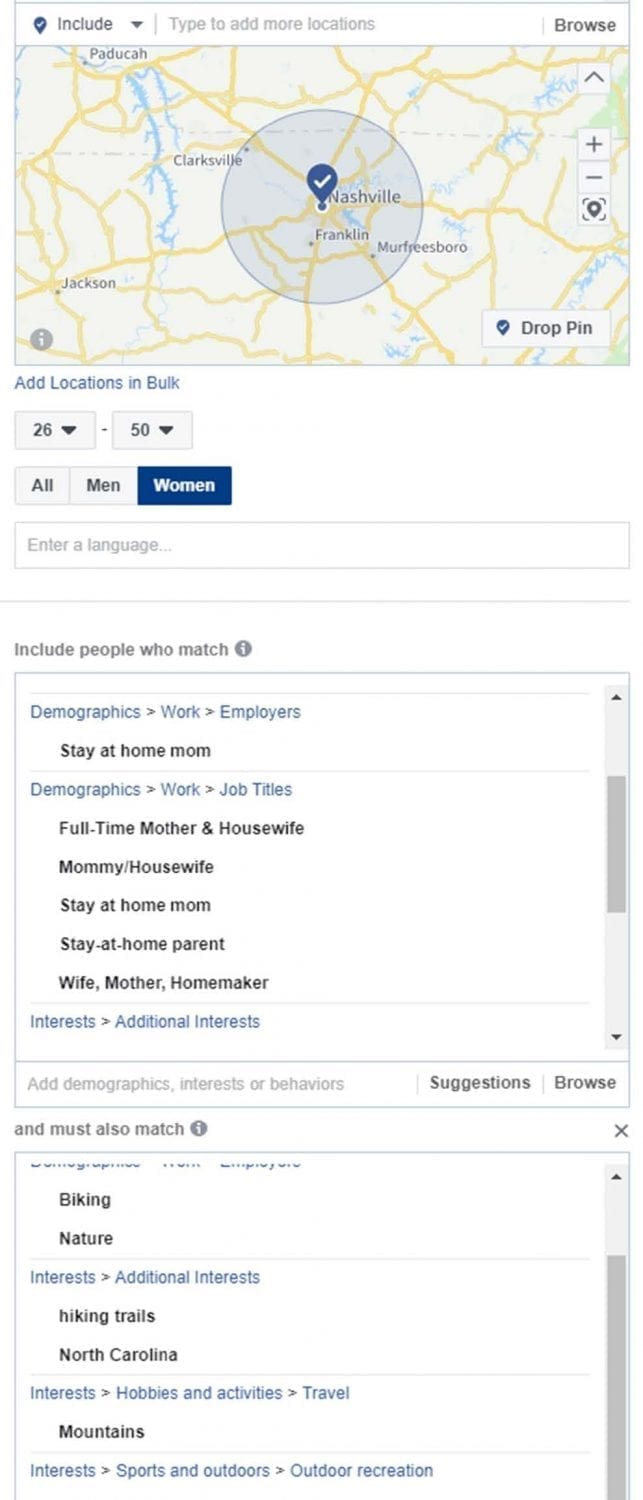The image is a detailed screenshot of a website interface designed to search for specific individuals within a defined geographic area. At the top left of the screen, there is a location icon followed by the word "Include" and a dropdown arrow. To the right of this, there is a field where users can type to add more locations, and in the far right corner, there is a "Browse" button.

Just below this section, a map is displayed with the city of Nashville highlighted. The map features a prominent light blue circle surrounding Nashville, indicating the selected area, along with a location icon marked with a white checkmark positioned over the city.

Below this map, there is an option labeled "Add location in bulk" and a dropdown menu indicating the age range "26 to 50". Beneath this, there are selections available to "Select all", "Select men", or "Select women". For this instance, the option to search for women has been chosen.

Further down, there is a search bar labeled "Enter a language." Following this, there is a section titled "Include people who match" which includes various demographic options to narrow down the search. These options include work-related criteria like employers and job titles, specifically targeting groups such as "stay at home mom", "job titles: full time mother and housewife", and descriptions like "mommy, housewife, stay at home parent, wife, mother, homemaker."

Additionally, users have the ability to add specifics under "Add certain interests or additional interests." This section allows for further filtering by demographics, interests, or behaviors. Users can choose to look at suggestions or browse through additional interests. Currently, some of the listed interests include "biking, nature, hiking trails, North Carolina," and "mountains."